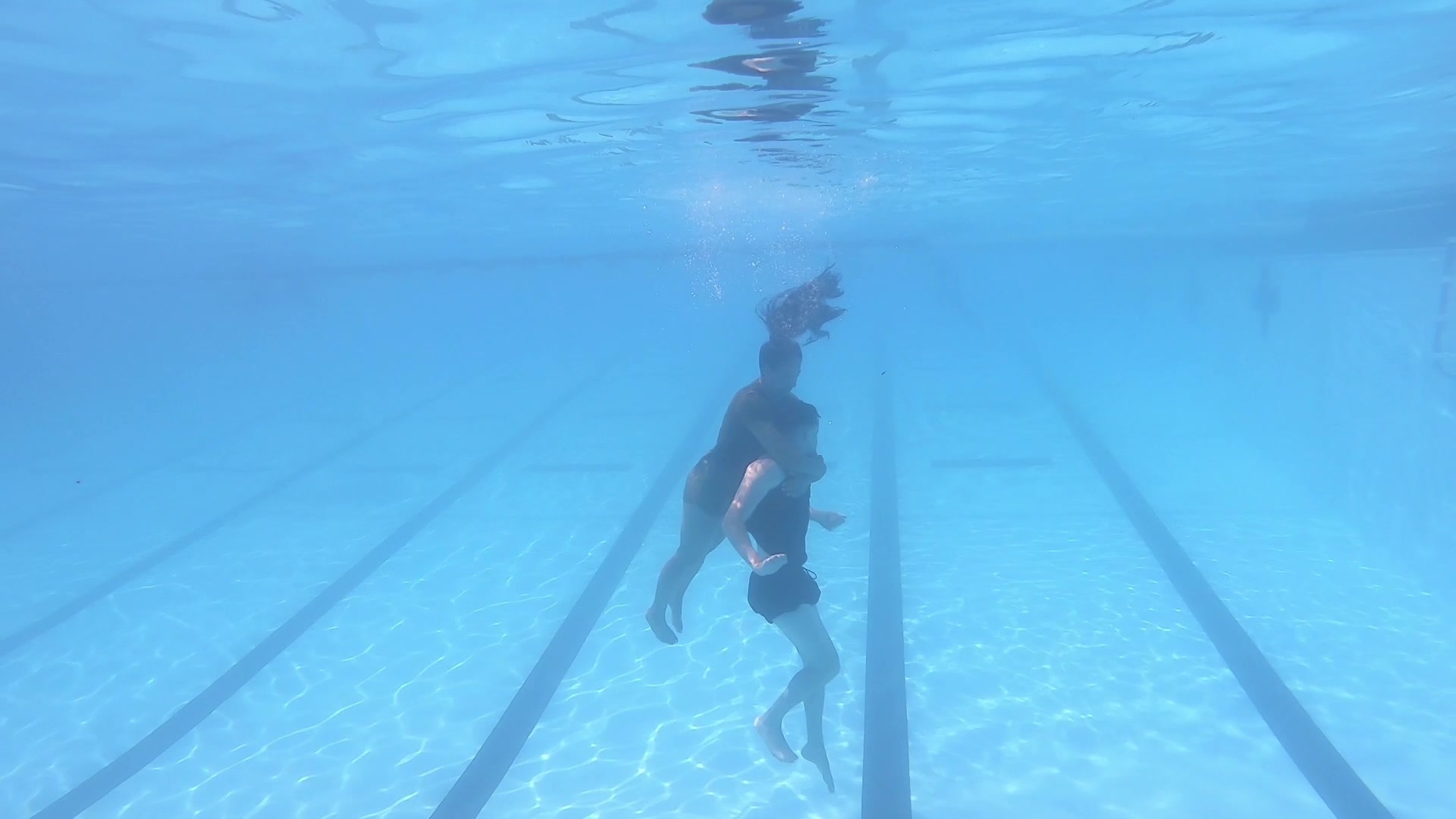The photograph captures an underwater scene in a deep, Olympic-sized pool. The entire image is suffused with a bluish tinge due to the water, giving everything a serene, aquatic hue. The pool's bottom and walls are a stark white, punctuated by black stripes and rectangles that delineate its lanes. Near the center of the image, two people, likely women, are submerged. The woman behind has long, floating black hair and is holding onto the neck of the person in front of her, creating a dynamic yet tender moment as if rescuing or supporting them. The top portion of the image reveals the underside of the water surface, reflecting the figures below. The scene is indoor, as indicated by the subdued lighting, adding a dramatic undertone to the composition.